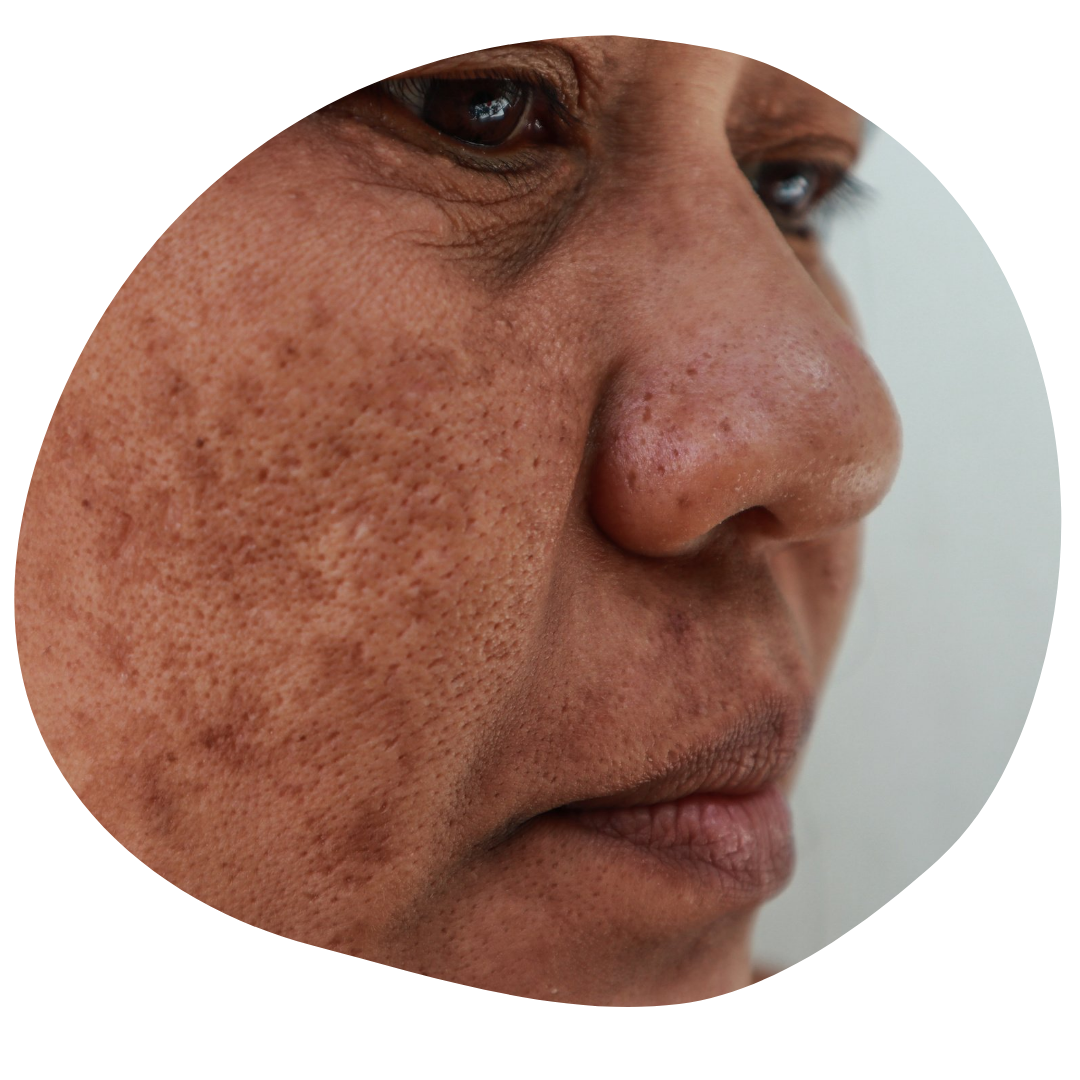This close-up image captures a middle-aged person with light to medium brown skin, presented in a circular vignette format. The individual is shown in a three-quarter profile, facing the viewer's right. The background appears to be either white in a dark room, gray, or slightly bluish. The person's eyes are a dark brown with noticeable small pupils, set beneath visible dark circles. Their face features distinct areas of discoloration, including age spots, rosacea, and signs of past acne or blackheads, with visible pores and indents on their cheeks and prominent smile lines. The skin tone appears darker brown with a reddish tint on their cheeks. The nose is wide and prominently displayed, while the lips bear some natural dark coloration on the outsides. The individual seems to be wearing minimal makeup, potentially a bit of natural-looking lip liner and black eyeliner, although the eyelashes appear thin. The overall photo focuses on the person's eyes, nose, one cheek, and lips, omitting the chin and hair.